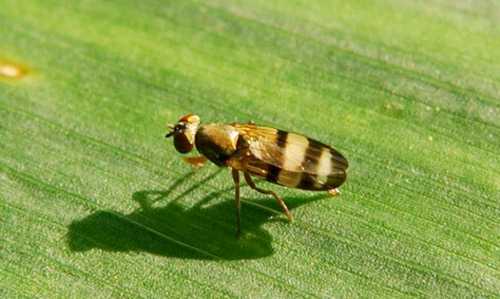In this highly detailed, close-up photograph, we see a small, unidentified bug, possibly a wasp or a bee, standing on a green leaf. The bug is characterized by its black and yellow striped thorax, two large compound eyes, two small antennae, and two transparent wings folded over its back. It appears to have six legs and is showing off a slender connection between its thorax and abdomen. The leaf underneath features distinct horizontal and diagonal stripes in various shades of green. A notable yellowish blemish, possibly a burn or stain, appears on the upper left-hand side of the leaf. The bright sunlight has cast a shadow of the bug that stretches towards the bottom left of the frame, nearly doubling its size. The photo's extreme zoom highlights the intricate textures of the leaf and the detailed patterns on the bug's body, creating a mesmerizing snapshot of nature.